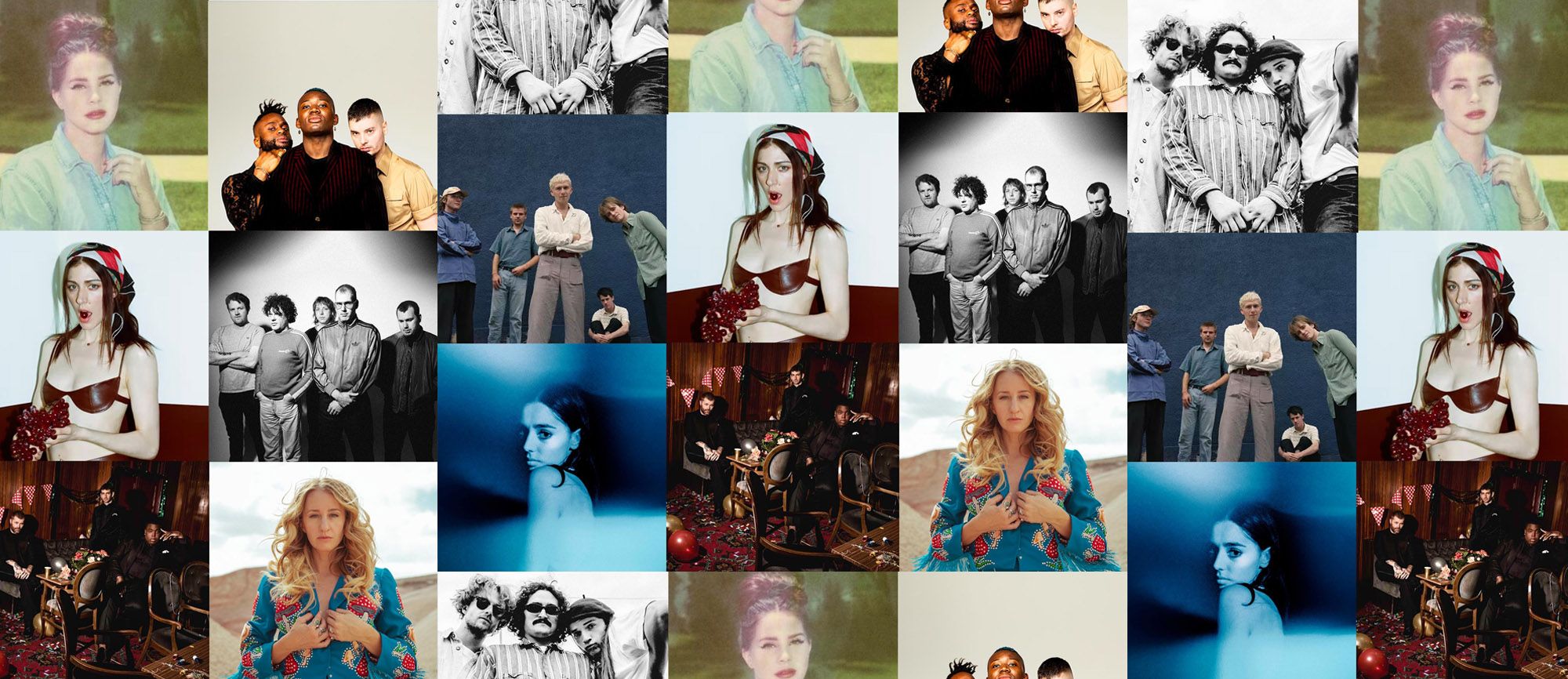A vibrant rectangular collage features approximately 13 photographs of young individuals, predominantly female, presented in various poses and settings. The images, which appear to be inspired by album covers, include both color and black and white portraits. Central to the collage is a striking image of a woman wearing a black bikini top and a bandana, staring directly at the camera. Surrounding her are varied images such as a blonde woman standing in a daylight desert scene, and another black and white portrait of a young woman with her back and shoulders exposed. The collage also repeatedly showcases a woman with a bun and red lipstick, a woman in a red bra, and several groups of men either sitting in what seems to be a living room or posing outdoors, giving an impression of musicians or bands. Additionally, a lady in a blue, long-sleeved shirt adorned with red and yellow flowers, set against a mountainous backdrop, appears at intervals. The photographs, meticulously placed without any spacing, are repeated in rows, creating a rhythmic pattern that emphasizes the ensemble's youthful and lively aesthetic.